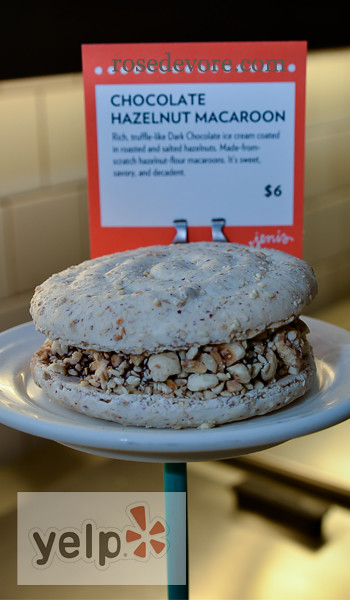The image showcases a delicious dessert displayed as part of an advertisement on Yelp. Positioned in the bottom left corner, there is a transparent white rectangle with the Yelp logo, featuring black lettering and a brown flower petal-like symbol. The central focus is on a white plate holding a sumptuous dessert labeled as a chocolate hazelnut macaron, priced at $6. The macaron consists of two white cookie layers sandwiching a rich, dark chocolate truffle center embedded with crushed hazelnuts. Behind the plate, a red sign with white and black text provides more details about the treat, describing it as featuring "rich truffle-like dark chocolate" and highlighting the dessert's sweet and savory decadence. Above the description, the sign bears the name "rosedivore.com" in light brown lettering, emphasizing the source of this enticing confection. The background is a white-tiled wall, slightly out of focus, bringing the dessert into sharp visual prominence, enticing viewers with its luxurious appearance.